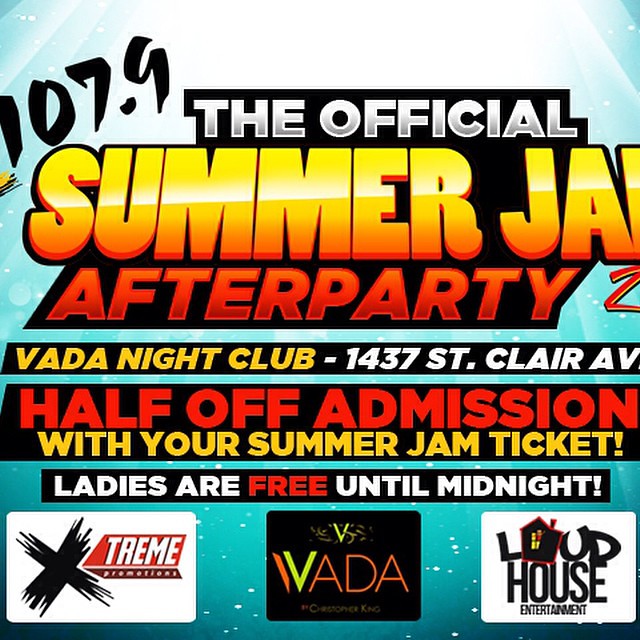The image is an advertisement for the official Summer Jam After Party 2, hosted by radio station 107.9. Dominating the top section, the words "Summer Jam" are in big, bold yellow letters, though the "M" is partially cut off. The event takes place at Vada Night Club, located at 1437 St. Clair Ave. Notable details include a half-off admission offer with your Summer Jam ticket and a special note that ladies are free until midnight, with the word "free" highlighted in orange. At the bottom of the image, three sponsor logos are featured: Extreme Promotions, Vada Nightclub, and Loud House Entertainment, with the "O" in Loud House shaped like a house. The background transitions from dark blue to aqua blue with a central area of white lighting, adding vibrancy to the announcement.